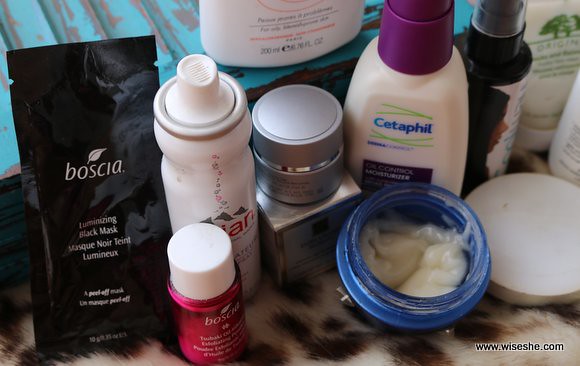This photograph showcases a collection of eight skincare products meticulously arranged on a table draped with a plush, leopard-print fabric. The products are neatly displayed, suggesting a bathroom or vanity setting. In the forefront, there is a black bag from the brand Boscia, spelled B-O-S-C-I-A. Next to it, there is a smaller product from the same brand, housed in a red container resembling either a lipstick or nail polish bottle. An Evian spray bottle sits prominently, followed by a smaller gray jar situated below a blue jar, which is open and reveals a white, gooey substance inside. A distinct plastic bottle of Cetaphil, marked with a red or maroon cap, stands out among the collection. Additionally, there are two other bottles: one black bottle and another bottle positioned on a stand, both adding to the diverse array of skincare products in the image.